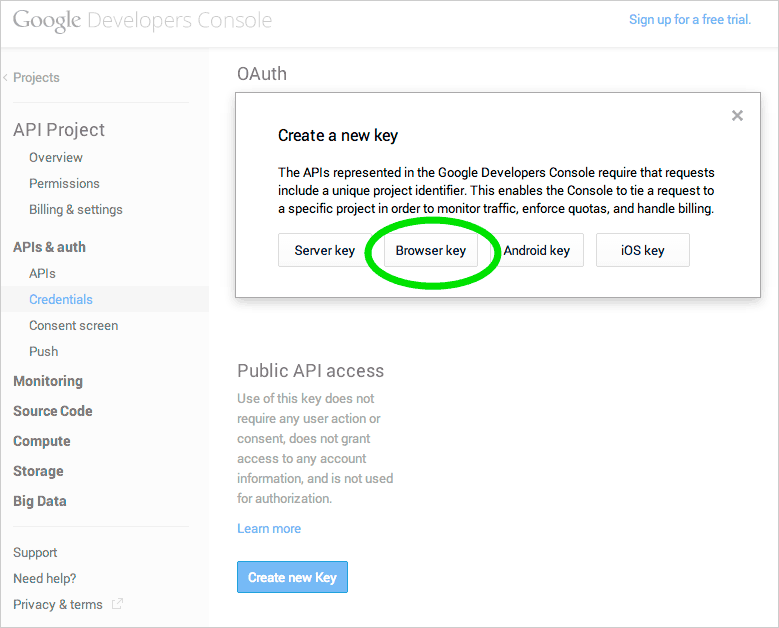This image depicts the Google Developer Console interface, specifically showcasing the "Credentials" section. At the top of the interface, a white navigation bar displays an option labeled "Sign Up for a Free Trial" in blue text on the right. On the left side of the navigation bar, there's a small label indicating "Projects," accompanied by a left arrow suggesting a dropdown or expandable menu.

The left sidebar enumerates various project management options such as "API Projects," "Overview," "Permissions," "Billing and Settings," "APIs and Auth," "Credentials," "Consent Screen," "Push," "Monitoring," "Source Code," "Compute," "Storage," "Big Data," "Support," "Need Help," "Privacy," and "Terms." The currently active section, "Credentials," is highlighted in blue, while the rest of the options are in a muted black or gray font.

Central to the image is the "OAuth" section where a pop-up window is visible with the title "Create a New Key." This pop-up explains that APIs enlisted in the Google Developer Console necessitate the inclusion of a unique project identifier. This identifier aids in associating requests to a specific project, facilitating traffic monitoring, quota enforcement, and billing management.

Displayed below this explanatory text, four key options are listed: "Server Key," "Browser Key," "Android Key," and "iOS Key." Notably, the "Browser Key" is circled in green, presumably highlighted using a photo editor for emphasis. All key options are stylized with white icons, gray outlines, and black text. This screenshot seems to have been taken for training or educational purposes, likely intended to instruct users on how to navigate and utilize the Google Developer Console effectively.